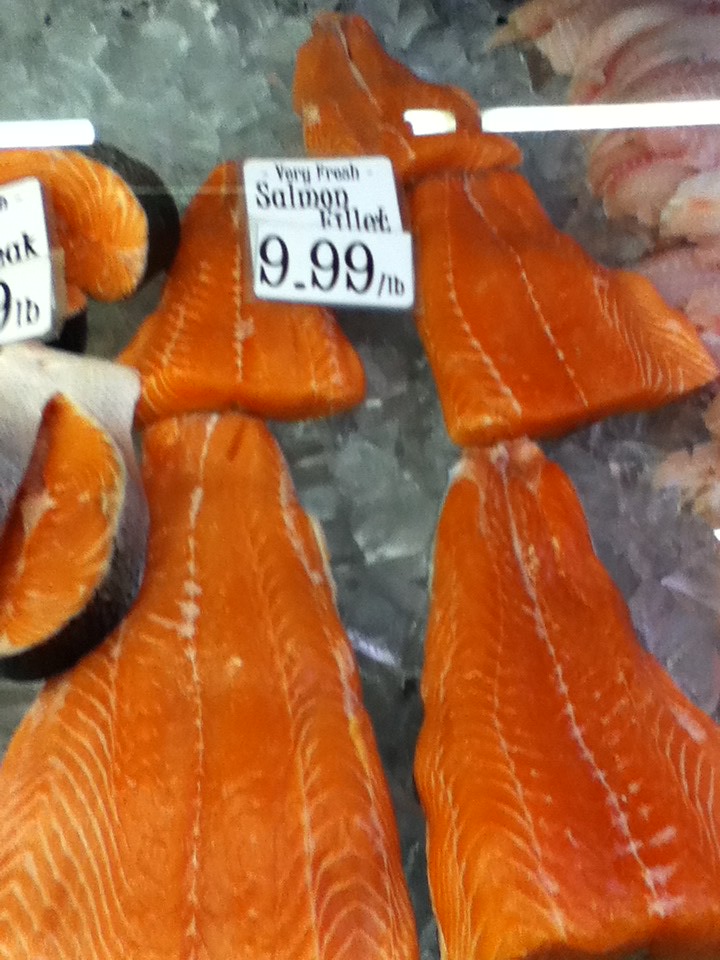This image depicts a neatly arranged seafood display at what appears to be a fish market or grocery store. Prominently featured are five meticulously cut salmon fillets laid on a bed of ice, their vibrant orange color accented by the white streaks of fat and muscle running horizontally. Behind the glass counter, these fillets are showcased to appear as fresh and delicious as possible. A white label above them reads "very fresh salmon fillet" and "9.99 per pound," indicating a more reasonable price likely from a time before significant inflation. On the left side of the display, two salmon steaks with their silvery skins catch the eye, while on the right, whiter fish fillets add variety to the array. The entire scene is illuminated by overhead fluorescent lights, whose reflections can be seen on the glass covering the display. The ice chunks beneath the seafood not only enhance the freshness but also create a crisp presentation of the various offerings.